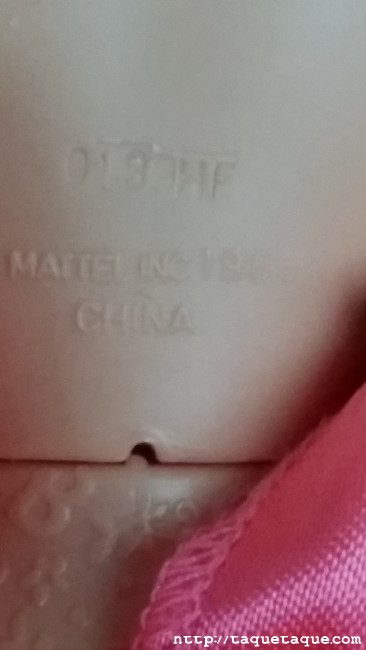In this close-up image, the upper two-thirds showcase a white plastic surface, possibly part of a toy, prominently featuring molded inscriptions in bas-relief. The text "Mattel Inc 19" is clearly visible, with "China" situated just below it. Above these inscriptions, there seems to be a stamped marking, likely reading "1HH" or "HF," though it's somewhat difficult to discern. The plastic surface includes a small, semi-circular cutout at its bottom edge, leading to another similarly colored plastic piece below, separated by a distinct seam with a tiny half-circular cutout. This lower plastic section features a raised pattern, including the number "8" or possibly a sideways "B," alongside several flower motifs. In the lower right-hand corner, there's a piece of pink cloth, appearing either coarsely woven or simply detailed due to the extreme zoom, allowing the individual threads to be seen, with a slight sheen and a visible highlight. At the very bottom of the image, a watermark reads "http://TechCadillacue.com."